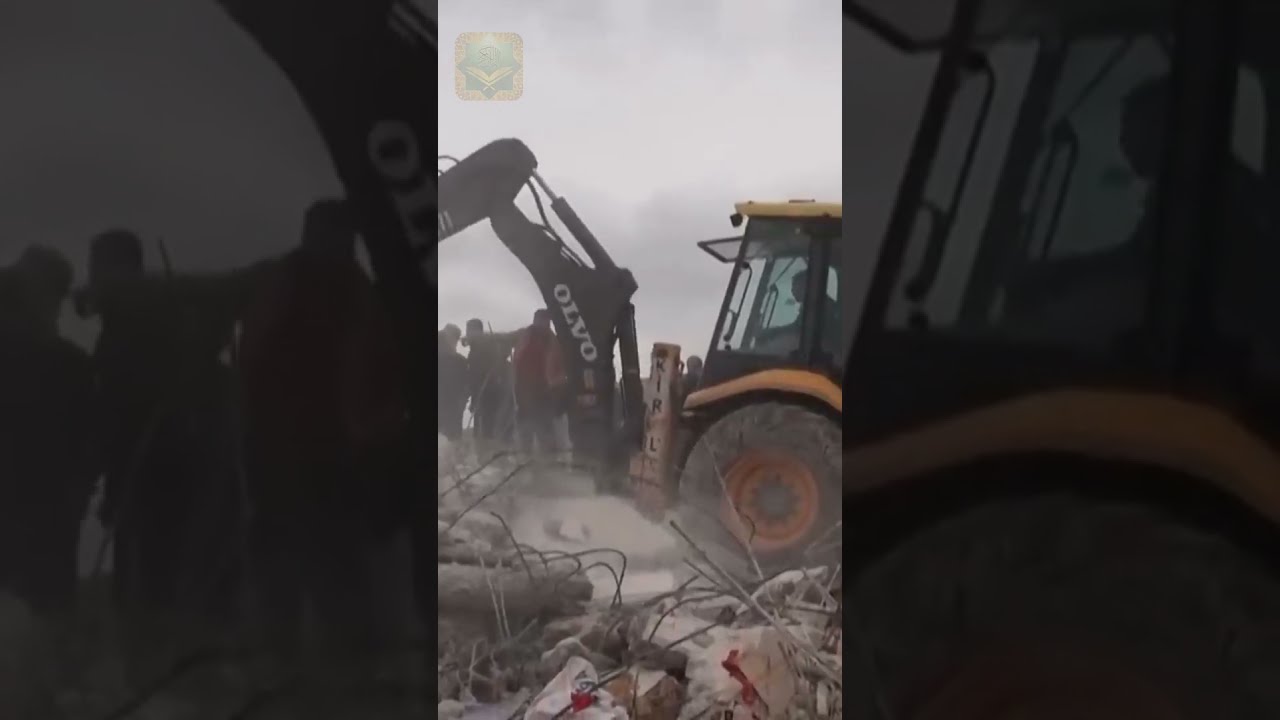This color photograph captures a dynamic construction site featuring an orange Volvo excavator with a crane attachment. The machine, equipped with large black rubber tires, is maneuvered by a driver visible within the glass-enclosed cab. Surrounding the vehicle are multiple onlookers; one individual is prominently pointing, seemingly directing the operation. The site itself is filled with rubble, including piled logs, concrete with exposed rebar, and other debris indicative of demolition work. The air appears hazy, possibly from dust or overcast weather, adding a dramatic effect to the scene. The photograph, likely a screenshot from a video, shows the midway action of the site, set against a gray, clouded sky.